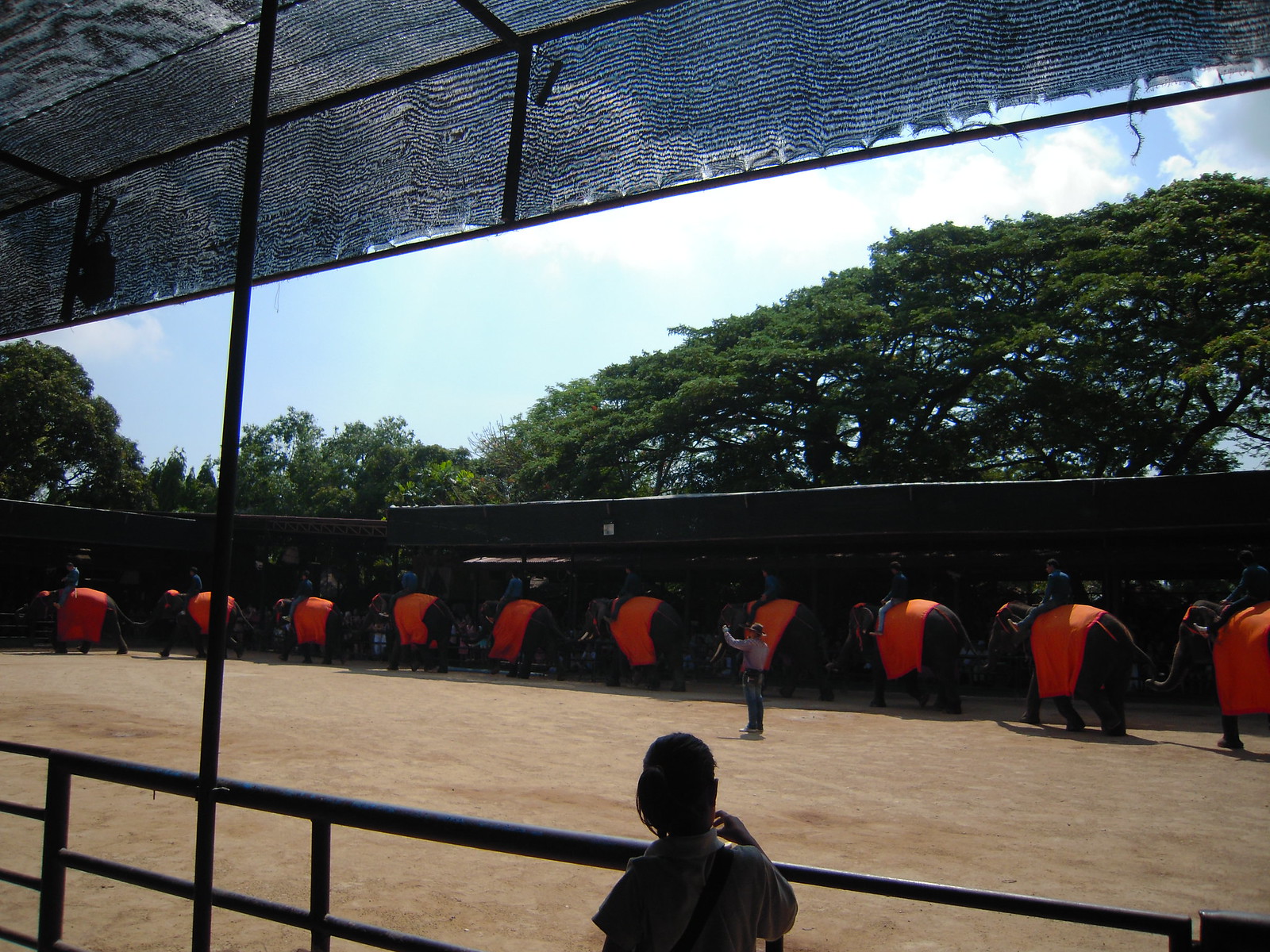In this photograph, we see a sandy, gravel-covered arena that resembles those used for horse shows or rodeo events. Encircled by metal railings and shaded by a black cloth awning, spectators can either stand or sit in the shade. The center of the arena is occupied by a train of around 10 or 12 young Indian elephants, each adorned with bright orange blankets draped over their backs. The elephants are walking in single-file, each one gripping the tail of the elephant in front with its trunk. Seated on the shoulder areas of these elephants are men, dressed in light blue jeans and dark blue long-sleeved shirts. Shadows cast over the elephants make their coloring appear dark brown. Behind the elephants, a wall separates them from some visible trees. A little girl with a ponytail and wearing a white short-sleeved shirt with a bag strap over her shoulder stands in the foreground near the railing. Also visible is a man in the middle of the arena, sporting a cowboy hat, long-sleeved shirt, and jeans, seemingly directing the elephants’ movement.